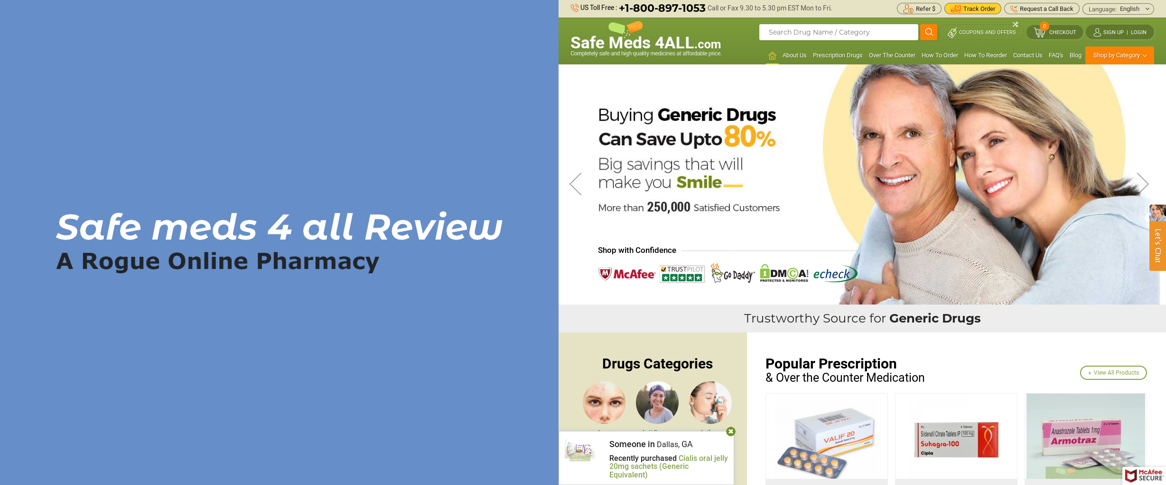This is a website with an easy-to-read layout. The left side prominently features a purple-blue image with the bold text "Safe Meds 4 All Review" in white, centering the phrase "a rogue online pharmacy." On the right side of the page, there is an image of a couple, with the woman affectionately wrapping her arms around the man. The caption next to them reads, "Buying generic drugs can save up to 80%, big savings that will make you smile," and highlights "more than 250,000 satisfied customers."

Below this section, badges from McAfee and GoDaddy are displayed, emphasizing that users can "shop with confidence," further endorsing the site's credibility as a trustworthy source for generic drugs. The website showcases various drug categories, accompanied by an image featuring three different people. It also highlights popular prescription and over-the-counter medications with images of various medication boxes.

At the top of the site, a banner includes an 800 number for customer inquiries, a search bar labeled "safemedsforall.com," and an additional orange bar on the right side of the header. The shopping cart icon in this section features an orange circle, indicating that there are items already in the cart.